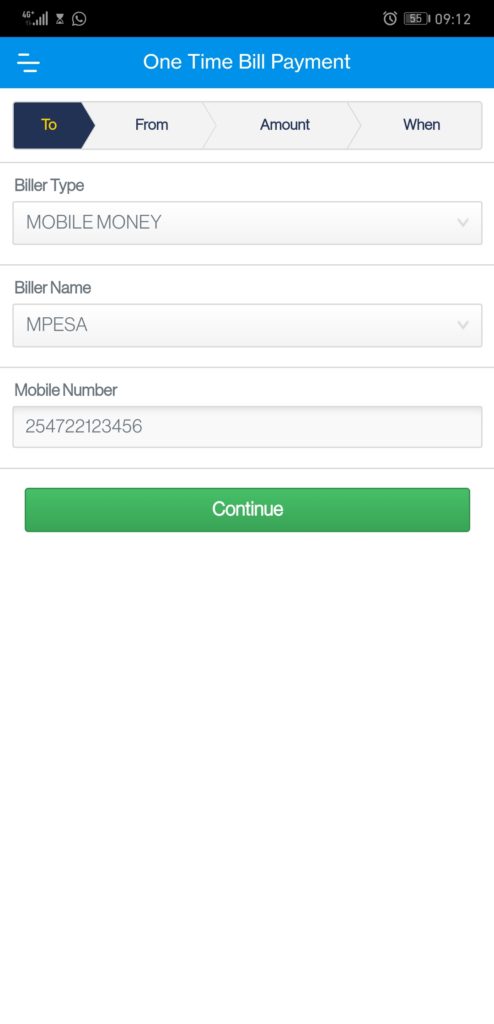The image depicts a cell phone screen with various interactive elements. 

At the top of the screen, there's a black strip featuring gray font that shows standard smartphone indicators: cellular signal bars, a timer indicating an ongoing phone call, an alarm icon, a battery percentage of 55%, and the current time displayed as 9:12.

Beneath this black strip, there's a blue strip occupied primarily by a vertical stack of three horizontal bars aligned on the left, suggesting a menu that can be accessed. The central text on this blue strip reads "One-time Bill Payment."

Progressing further down the screen, the interface displays labeled fields for bill payment details. In a gray strip marked "To," the tab is currently open to the "Biller Type" field, which is set to "MOBILE MONEY" in uppercase letters, with a dropdown menu available. Directly below, within another gray section, is the "Biller Name" field with "M-PESA" selected, also a dropdown menu.

Continuing downwards, the "Mobile Number" field contains the number "254722123456." 

At the bottom, a long, thin green button with the word "CONTINUE" in white text spans horizontally more than vertically.

The overall screen design uses a color palette of black, gray, white, blue, yellow, and green, with substantial white space at the very bottom, nearly matching the amount of occupied space at the top of the screen.